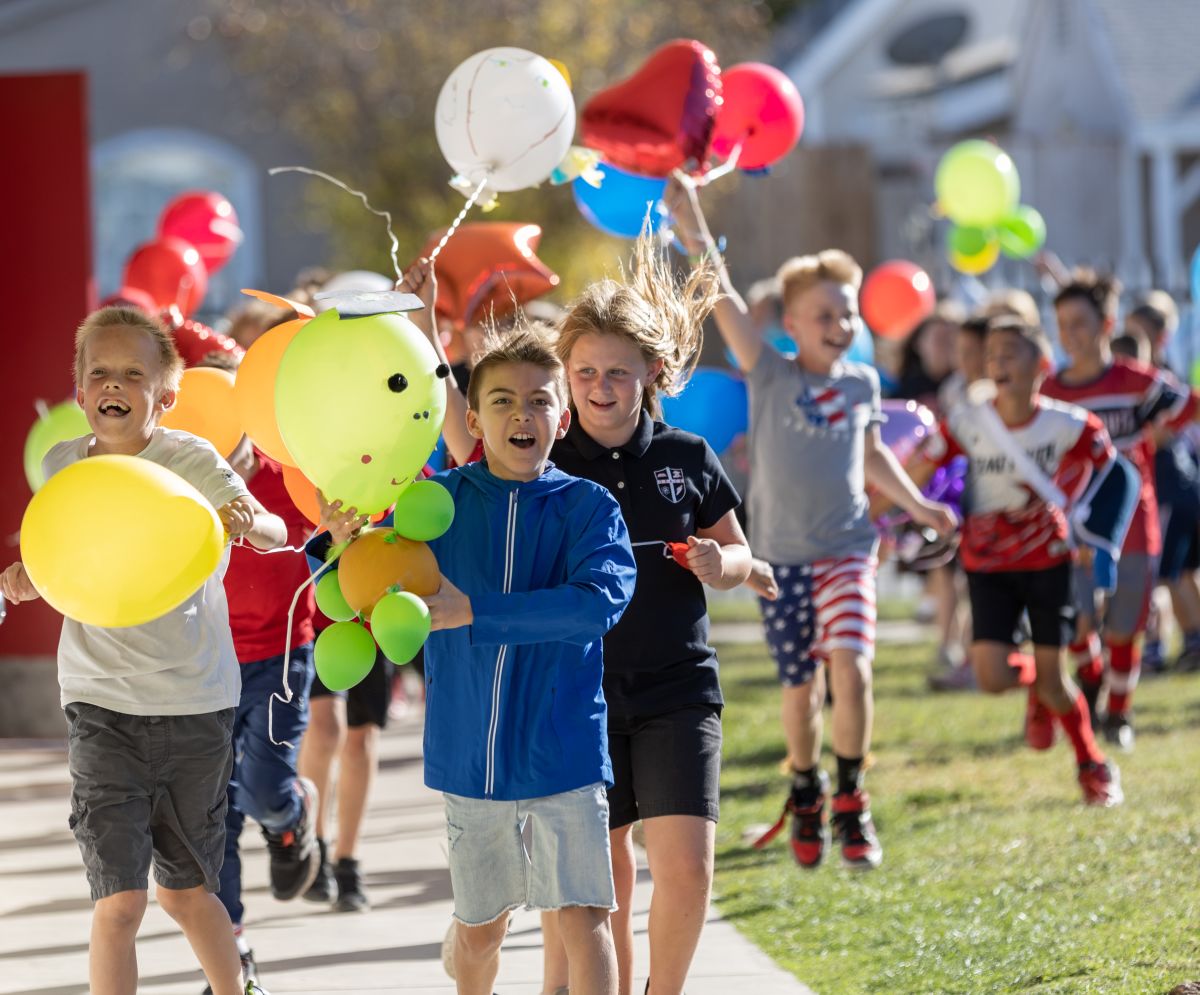The high-resolution photograph captures a lively scene of several dozen children, likely aged 10 to 11 years old, running energetically toward the camera. It's a bright, sunny day, evidenced by their attire of shorts, t-shirts, tennis shoes, and light jackets—typical for warm weather. The children, who appear to be predominantly Caucasian, display expressions of sheer joy and excitement. Each child clutches balloons of varying sizes, shapes, and vibrant colors, including green, yellow, red, white, blue, purple, and even copper. In particular, the closest boy to the camera is holding several balloons, one of which features a drawn-on face.

The scene appears to be set outdoors, possibly in a backyard or a school field, judging by the sight of concrete and grass underfoot. In the blurred background, the edge of a house and perhaps part of a motor home are visible, suggesting a casual, open-air environment. The event might be a celebration such as a birthday party, the end of the school year, a field day, or even a 4th of July festivity, as some children are adorned in red, white, and blue. Despite the various possible themes, the common element is the clear happiness and exuberance of the children, creating a joyful and heartwarming scene.